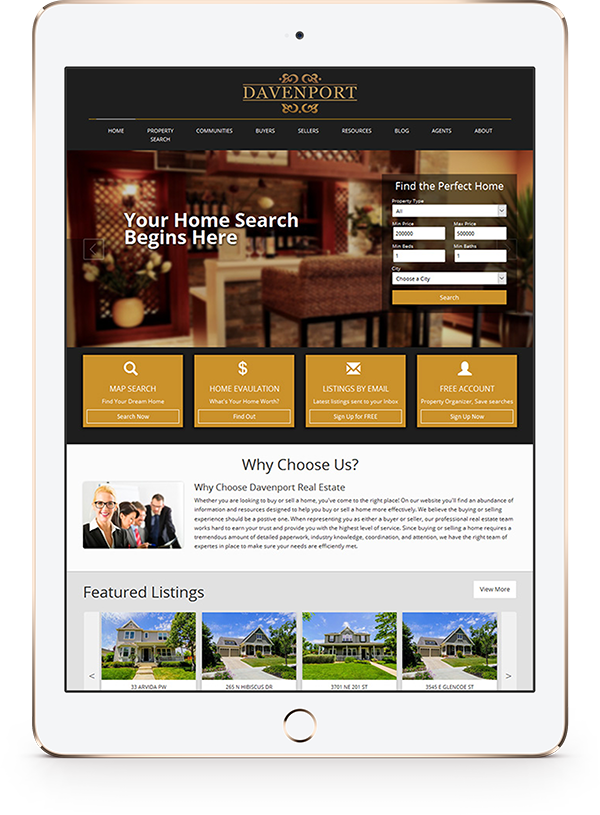**Website Interface Description: Davenport Real Estate Platform**

On the phone screen, the web page showcases the Davenport Real Estate platform. The interface features a sophisticated black border with elegant gold typography displaying the name "Davenport" prominently at the top. Beneath the name, a gold line provides a tasteful underline.

The navigation bar includes several key sections listed in gold letters: Home, Property Search, Communities, Resources, Blog, Agents, Buyers, Sellers, and About.

The main section of the page includes a slightly blurred image of a home interior with the text "Your home search begins here" superimposed on it, creating a welcoming focal point. 

To the side of this image, a user-friendly search bar is available, labeled "Find the Perfect Home." This feature enables users to filter options based on property type, price range, and desired city before hitting the search button.

Below this section, several additional options are provided: Map Search, Home Evaluation, Listings by Email, and Free Account.

Further down the page, a professional image captures a group of agents seated together, accompanied by the encouraging phrase "Why choose us."

The site's organized layout concludes with a "Featured Listings" section displaying four thumbnail images of select homes, enticing potential buyers with high-quality visuals of available properties.